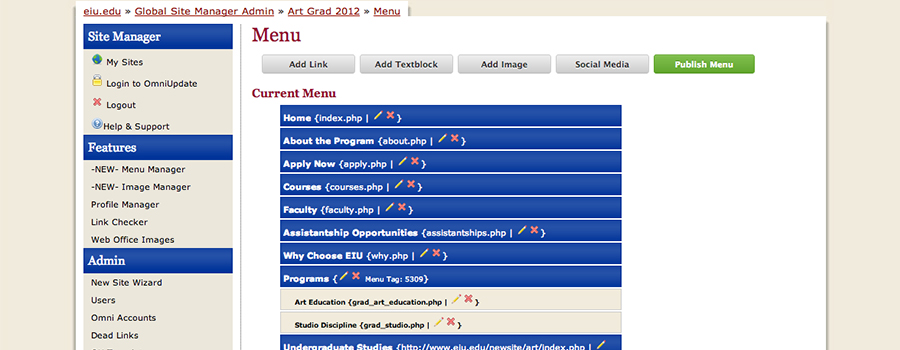In the image, the interface of a website editing platform under the URL "eiu.edu" is prominently displayed. At the top, there is a navigation trail marked by arrows leading through "Global Site Manager Admin," followed by "ArtGrad 2012," and ending at "Menu." Below this trail, the word "Menu" appears again, larger and more prominent, indicating the section being edited.

The main part of the interface showcases several interactive tabs and buttons, each labeled for its specific function: the leftmost tab reads "Add Link," followed by "Add Text Block," "Add Image," and "Social Media." To the right of these tabs is a striking green button labeled in white text, "Publish Menu." Just beneath this button, in stark red text, is the label "Current Menu."

The "Current Menu" section lists a series of blue squares, each with a corresponding link name and its associated file path:

1. Home - Index.php
2. About the Program - About.php
3. Apply Now - Apply.php
4. Courses - Courses.php
5. Faculty - Faculty.php
6. Assistant Opportunities - Assistantships.php
7. Why Choose EIU - Why.php
8. Programs

Beneath this list, in gray text, are additional categories such as "Art Education and Studio Discipline," accompanied by ".php" extensions, and a label for "Undergraduate Studies."

On the left side of the interface, navigation options are displayed in black text, listing sections like "Site Manager," "Features," and "Admin," which likely direct the user to other parts of the site management system. The entire layout provides a comprehensive overview of the web platform's site navigation and editing capabilities.